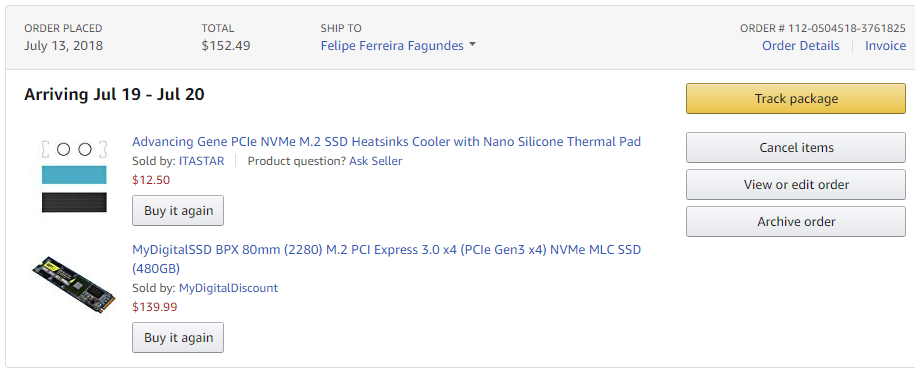Here is a detailed caption:

---

This partial screenshot from an Amazon order summary shows a purchase made by Felipe Ferra Fagundes on July 13, 2018, totaling $162.49. The order includes two items: an Advancing Gene PCIe Heat Sink Cooler with Nano Silicone Thermal Pad priced at $12.50, and an 80mm M.2 PCI Express SSD 480GB priced at $139.99. Both items were sold by different third-party sellers. The order status indicates that the items are still in transit, with an expected delivery window between June 19 and July 20. The screenshot also displays options to view order details, invoice, and track the package. Additionally, there is an option to cancel the items if necessary. The order number is visible on the top right of the screenshot, along with other pertinent details such as the inventory view.

---